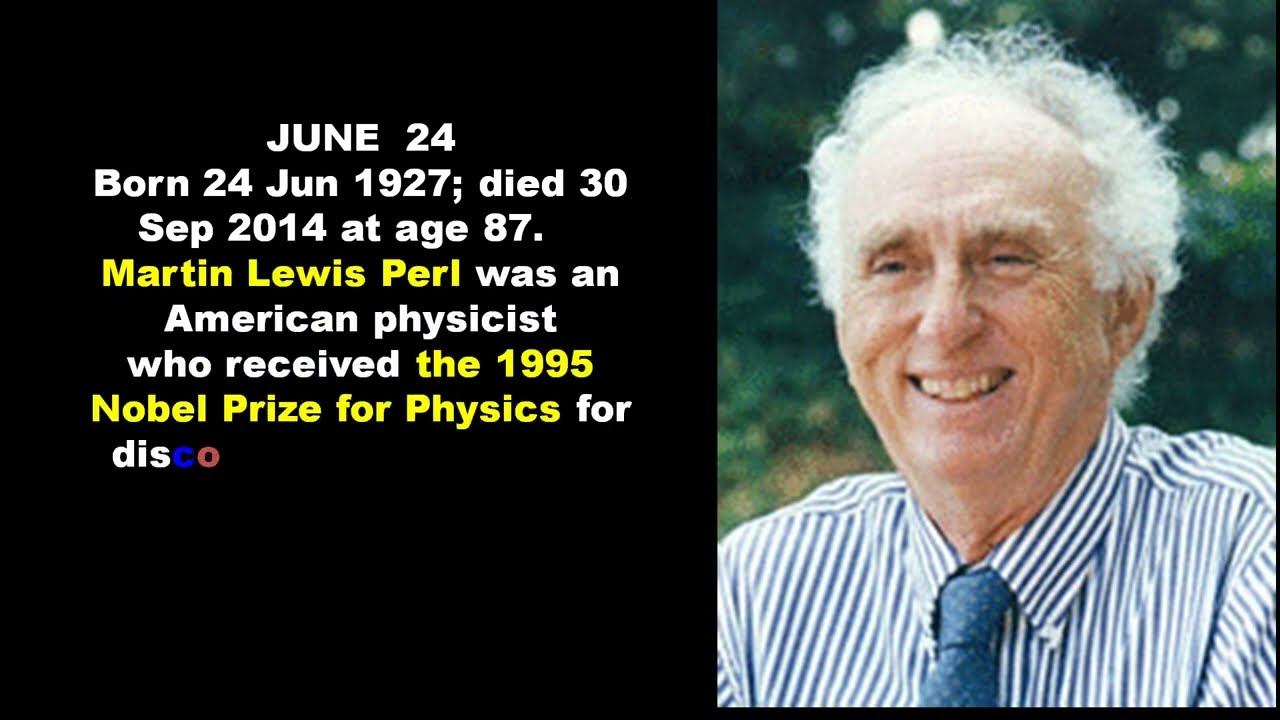The image consists of two sections: the left side features a black background with detailed textual information, while the right side displays a professionally taken photograph of an elderly man, identified as Martin Lewis Perl. Perl, an eminent American physicist born on June 24, 1927, and who passed away on September 30, 2014, at the age of 87, is best known for receiving the 1995 Nobel Prize in Physics for his discoveries. The text on the left includes a mix of colors: June 24, born 24 June 1927; died 30 September 2014 at age 87, all in white, while "Martin Lewis Perl" is highlighted in yellow. Below, in white text, it states, "was an American physicist who received," followed by "the 1995 Nobel Prize for Physics" in yellow. The word "for" is in white, and "disco" has 'DIS' in white, 'C' in blue, and 'O' in red, with the latter two letters smaller in size.

In the photograph on the right, Perl is depicted smiling and appears to be in his 70s or 80s, with a wrinkled face and frizzy, fluffy, white-gray hair. He is clean-shaven and donned in a blue and white striped button-down dress shirt accessorized with a blue tie adorned with a light-colored pattern. The background shows an outdoor setting on a sunny day with out-of-focus leaves, possibly from a tree or plant, adding a natural touch to the portrait.